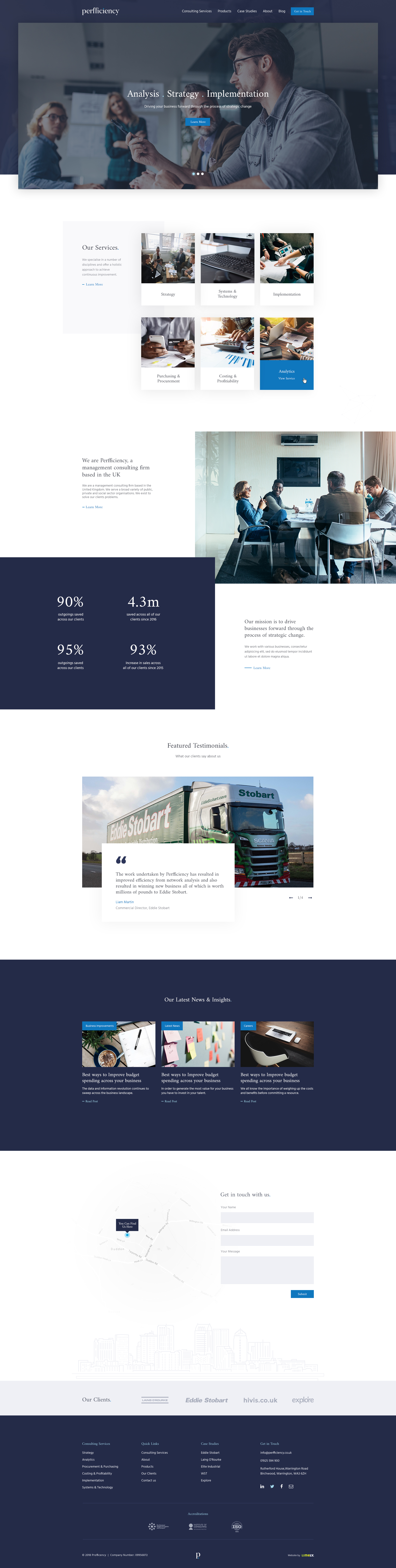The image appears to be a detailed screenshot of a corporate web page. At the top, the page features a heading related to "Analyze" or "Analysis Strategy and Implementation". Following this, there's a section titled "Our Services" showcasing six small images, although the specific headlines of these images are not discernible.

Below the services section, there's a large image depicting a group of people assembled in a meeting room. Adjacent to this image, a statistics box is visible, displaying figures such as 90%, 95%, 4.3 million, and 93%, though the context for these numbers is unclear due to the small text.

Further down, the page includes featured customer testimonials, highlighted by various quotes. Above these quotes, there's a photograph of a green and white Andy Stobart truck captured on a sunny day in a rural setting.

Additionally, the page features a segment with a blue background containing three thumbnails. These thumbnails display office-related images, including post-it notes, a desk and chair, and a writing pad with a pen.

Towards the bottom of the web page, there is a navigational footer with links to various sections such as Home, Contact Us, FAQ, and similar pages.